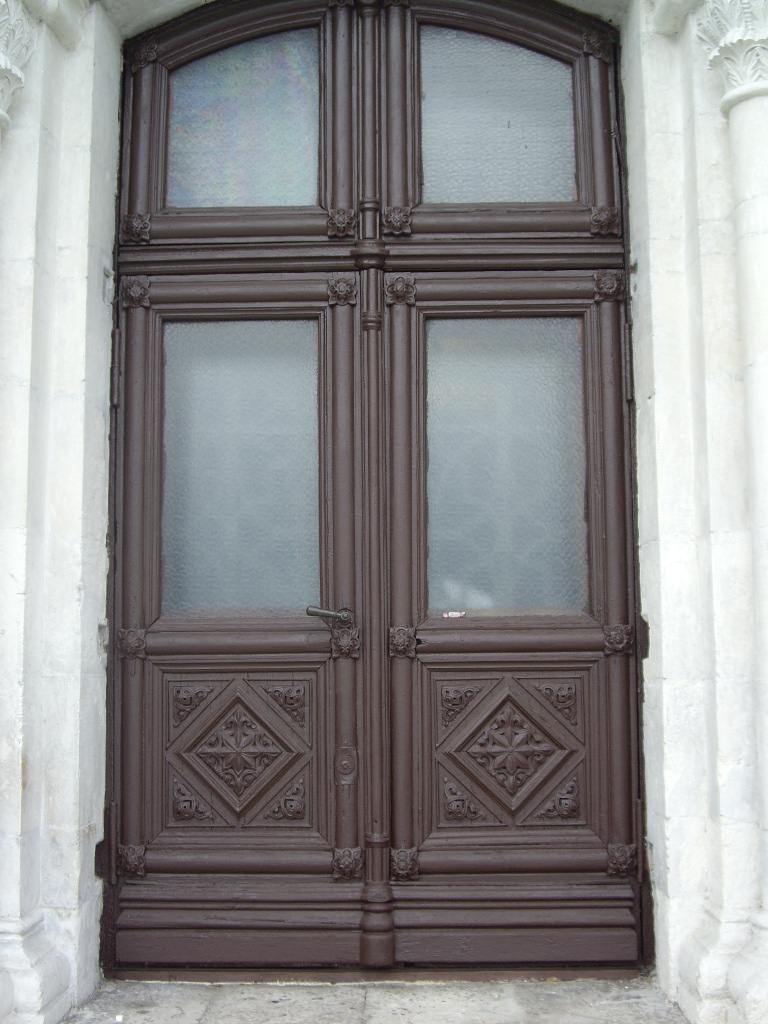The image showcases a substantial, tall, double-sided doorway with an industrial design. Each door, crafted in brown wood, features four small, foggy windows at the top, suggesting they do not open. The doors open symmetrically, from the center, and a gray handle is affixed to the left door. Detailed, outward metal designs frame these windows and the door edges, with each corner adorned with elaborate insignias.

The lower portion of the doors includes intricately engraved wooden sections, featuring rotated squares with layered, intricate patterns. The doorway is part of a tall, elegant building with a slightly run-down exterior. The structure is made primarily of white concrete, with a gray concrete entrance floor. Tall white columns stand prominently on either side of the doorway, enhancing the grand yet somewhat worn facade of what appears to be a historic or governmental building.